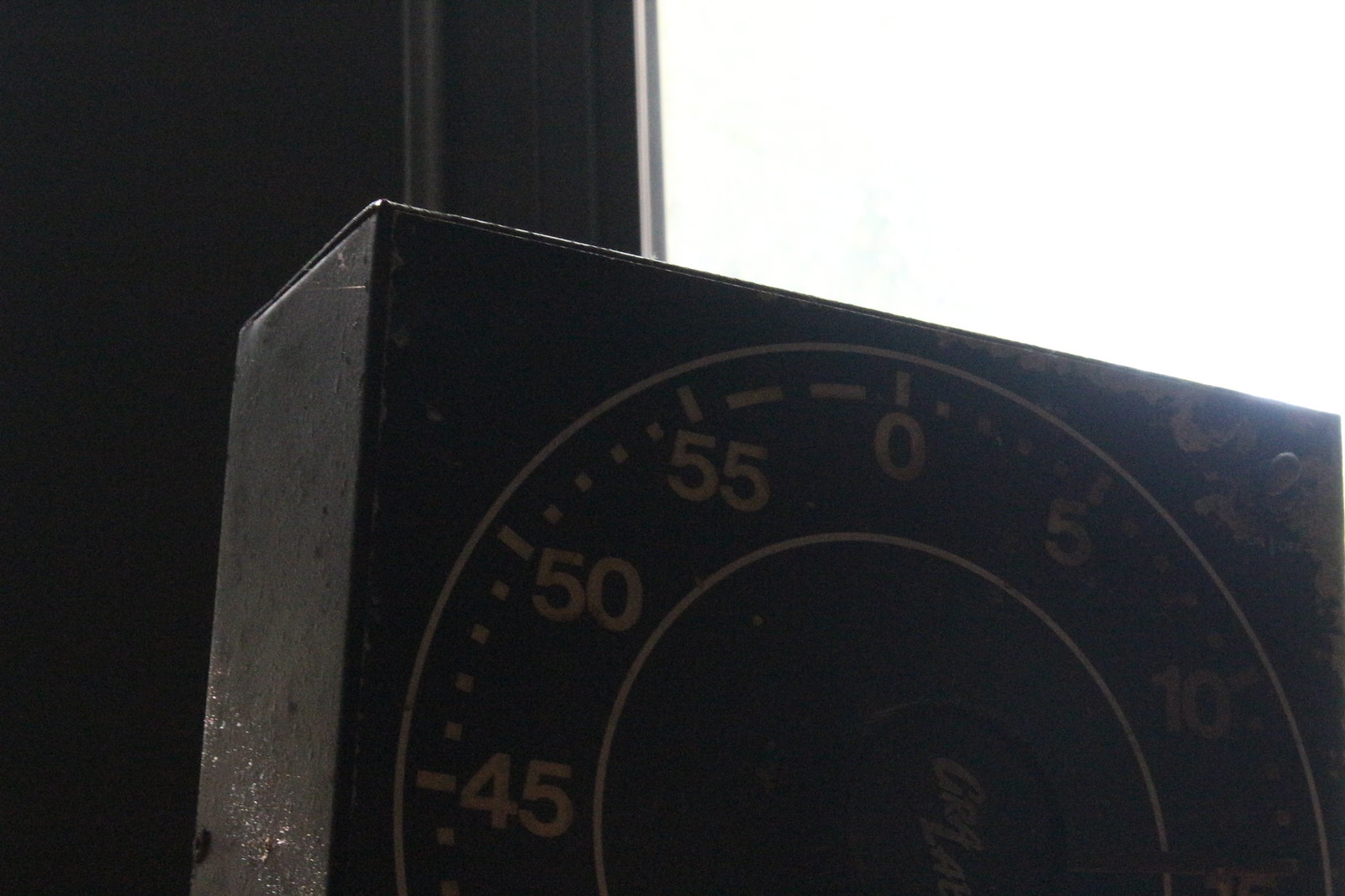The photograph features the top half of an intricately designed clock mounted on a dark brown wooden wall. In the upper right corner, the image is stark white, contrasting sharply with the upper left, which is dominated by a vertical black bar that stretches from top to bottom. Centered in front of this bar is a prominent black 3D rectangle, serving as the base for the clock’s display. The clock face itself consists of two concentric white circles encircling gold numerals that mark the minutes in 5-minute increments, ranging from 0 to 55. The number 0 is positioned at the top, and on the left side, the numbers 45, 50, and 55 are clearly visible. Notably, a word is inscribed in the center of the circles, though it is partially cut off and unreadable. The detailed craftsmanship of the clock and its sophisticated design are evident, creating an elegant yet functional piece against the wooden backdrop.